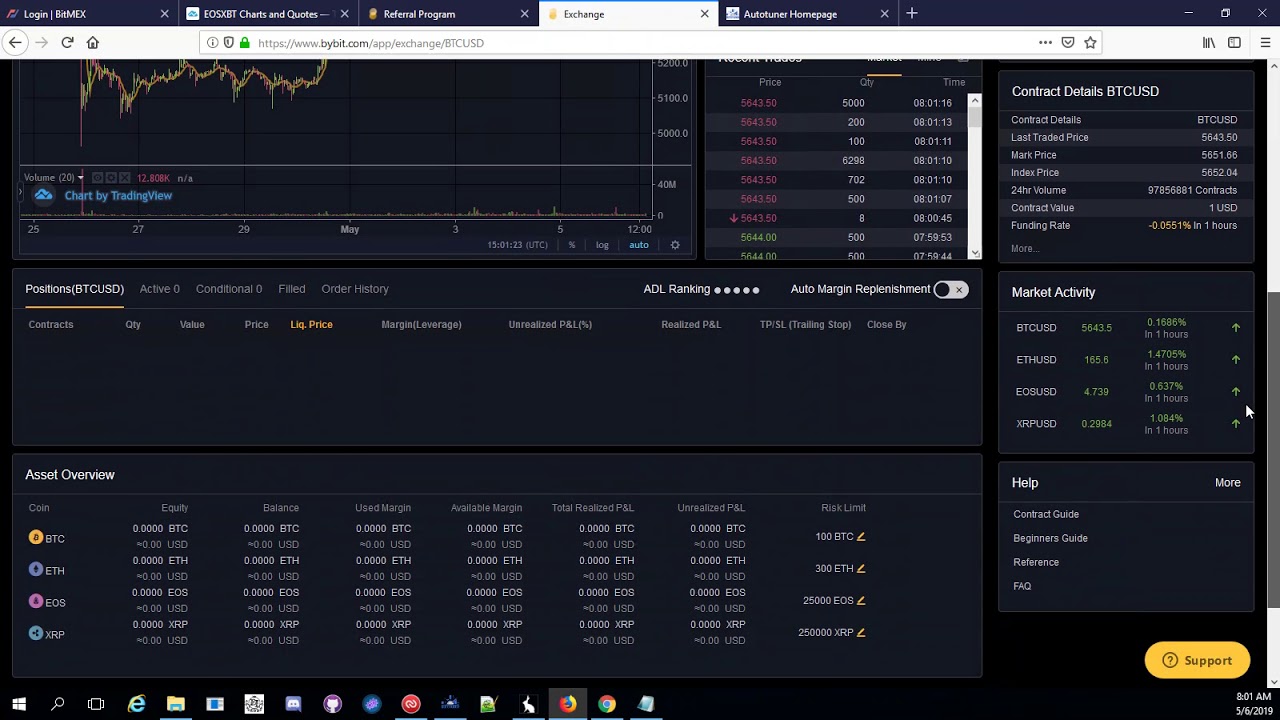The image depicts a vertically-oriented, rectangular user interface of a digital platform with very small and hard-to-read print. At the very top, there's a slim horizontal bar featuring clickable tabs. The visible tabs include "Login," "Chats," "Program," and "Exchange," the latter of which is currently active and highlighted in white. Another tab that possibly says "Homepage" is seen, whereas the remaining space in this line is blank. Below this top bar is a thin white rectangle serving as the URL address bar.

The main body of the interface is predominantly black, divided into various sections. In white text, partially visible labels such as "Postscript," "ADL Ranking," with a five-star rating graphic, "Auto Margin," and "Market Activity" can be seen. Additionally, there's an "Overview" section. At the very bottom of the interface, standard computer icons are displayed along with an orange oval button marked for "Support."